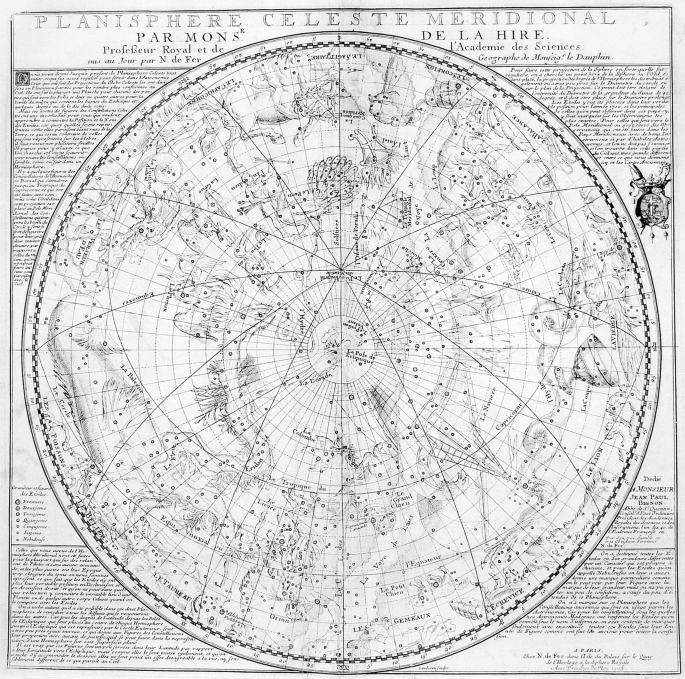This square, black-and-white image appears to be an old map or representation of the stars, titled "Planisphere Celeste Meridional." The map is encased within a thin black line border and occupies the entire frame, with textual details in the corners. The main feature is a large circle extending to the edges of the square, portraying a view from possibly the North Pole with radial lines that resemble latitude and longitude if it were Earth. The intricate design within the circle includes various lines and illustrations of constellations, though the details are faint and densely packed, making them difficult to discern. In the corners surrounding the main map, there is an abundance of tiny, detailed text. Notably, the upper left corner also features the words "Parmons," while the right-hand side includes the term "De la Hier." This detailed and elaborate illustration seems to depict a celestial map, likely used for observing the constellations.